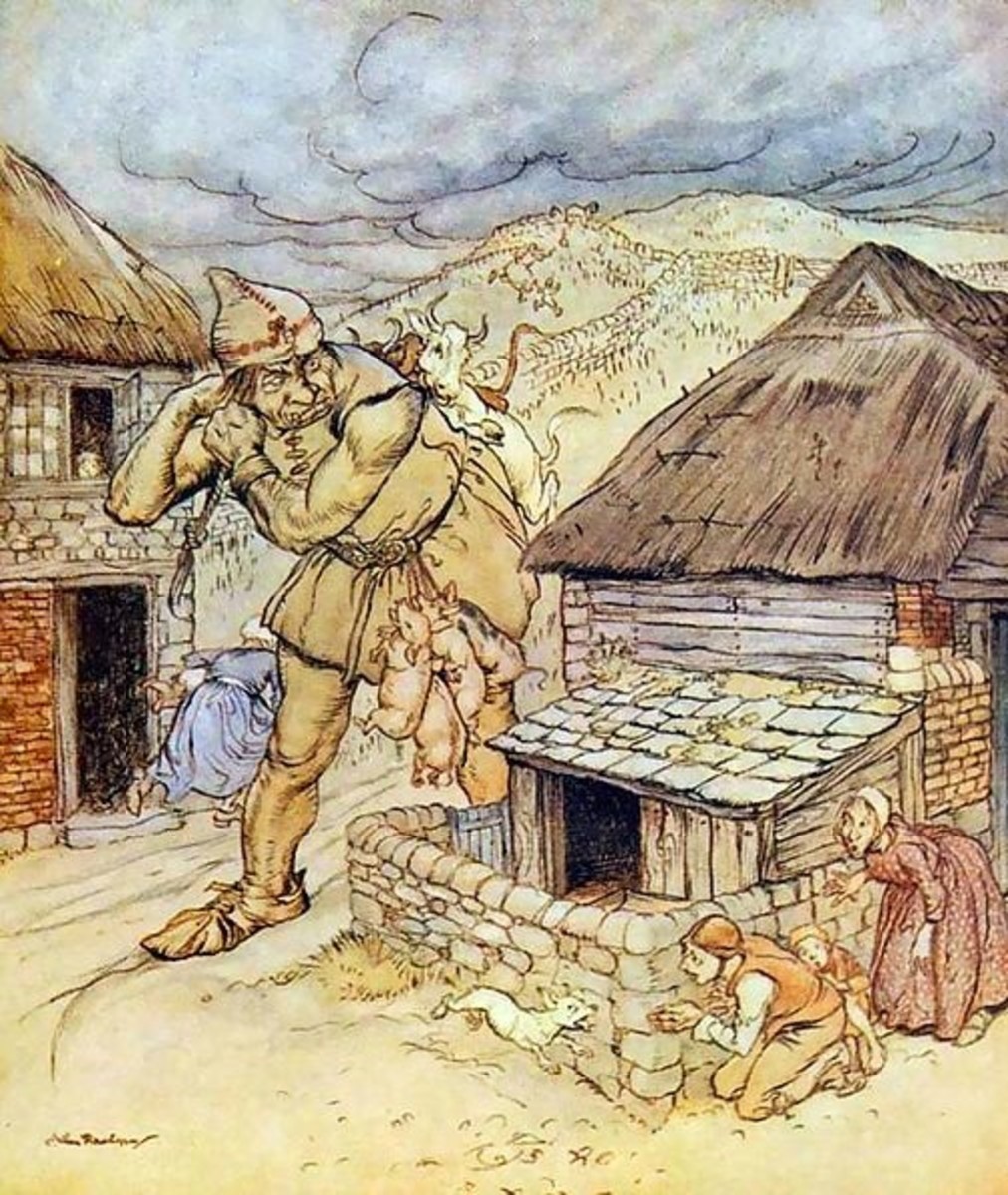This is a highly detailed line drawing, reminiscent of an old illustration from a vintage book, dominated by muted shades of yellow, tan, and red. The scene is set in an 18th-century farming village with medieval influences, characterized by thatched roofs and wooden slat walls. A menacing giant looms over the village, his form almost as tall as the rooftops. The giant is dressed in a rugged burlap smock, complete with crude, tied-together shoes and a pointed cloth cap, suggesting he has descended from the distant mountains.

The giant's face is ugly and angrily determined as he actively gathers the villagers' livestock. He has several cows roped over his shoulder and pigs, numbering anywhere from four to five, suspended from a sash around his waist. The villagers are in a state of panic; two women, dressed in simple attire — one in a white bonnet and red dress, the other in a white shirt, brown vest, and light brown pants — along with a child, hide in fear behind a cobblestone wall. They desperately try to call to a dog to keep it from the giant's grasp. In the background, another woman in a blue dress can be seen running away from a house, further emphasizing the chaotic scene. The style of this artwork resembles fantasy illustrations, with watercolor-like coloring and dark line art that provide definition, evoking an image straight from a classic King Arthur tale.